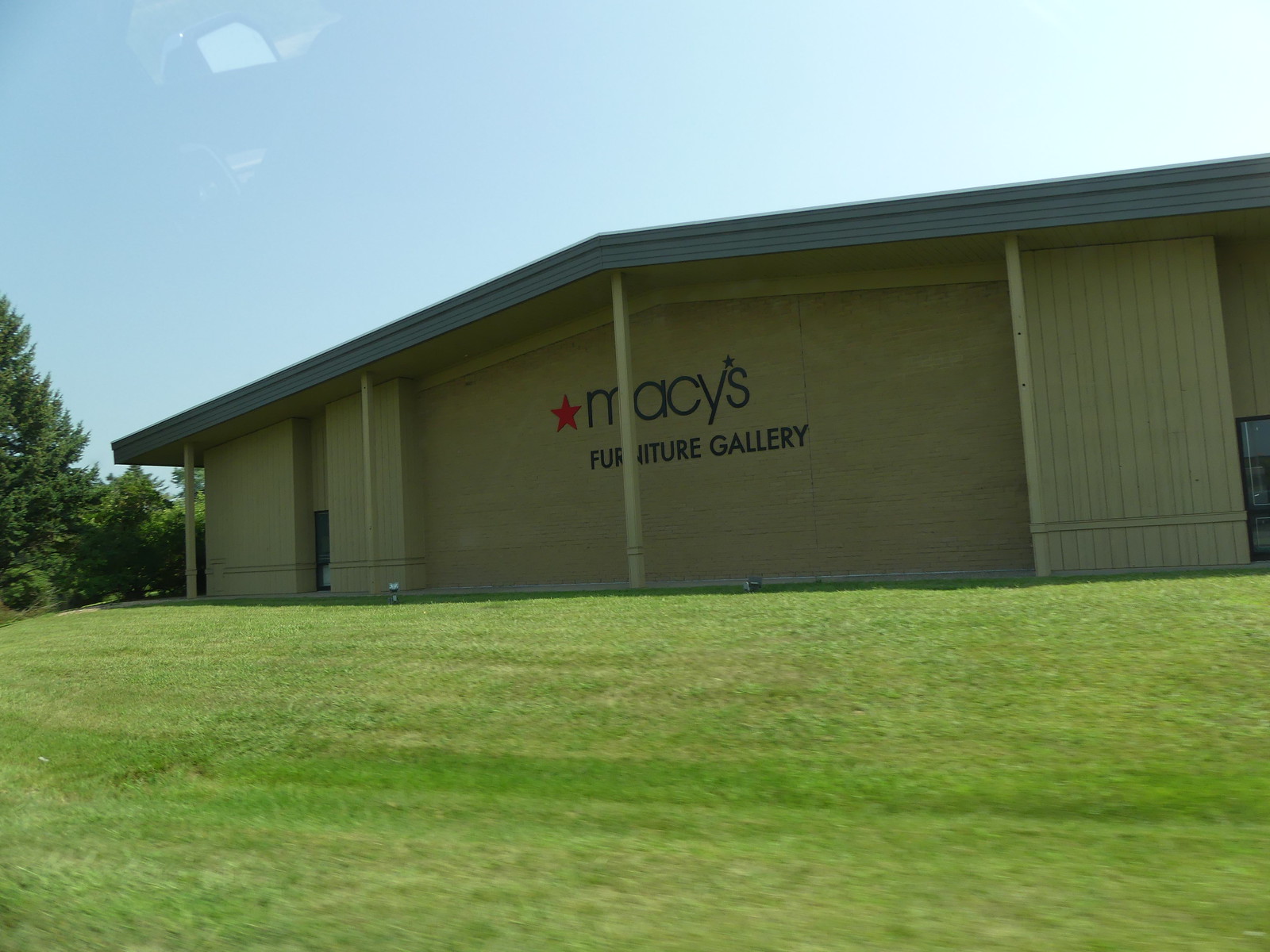A panoramic view of a Macy's Furniture Gallery, a specialized branch of the popular department store, featuring sophisticated and stylish interior furnishings. The photo captures the sprawling exterior of the establishment, which is surrounded by a meticulously maintained lawn, adding a touch of greenery to the upscale ambiance. The facade is modern and inviting, indicative of the quality and variety of home decor items and furniture pieces housed within. The bright, sunny day enhances the appeal, making the gallery look all the more welcoming and impressive.